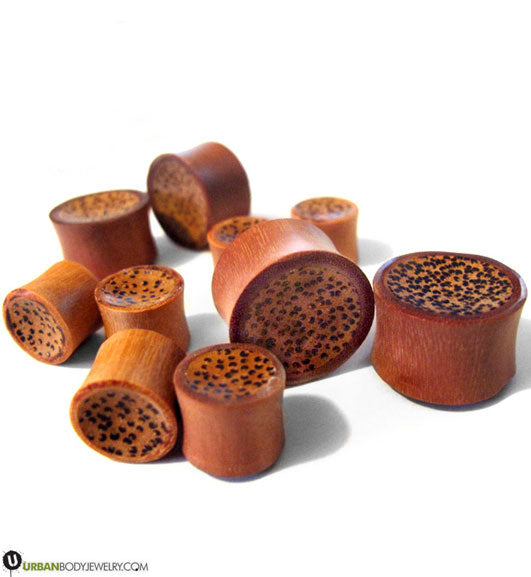The image features an assortment of cylindrical, can-shaped pieces of body jewelry resembling corks, scattered haphazardly on a white surface. These pieces, used for stretched earlobes, come in various sizes and shades of brown, from dark to tan, with natural wood-like grains and a speckled appearance on the top ends, possibly mimicking mold. Some of the cylinders are upright while others are laid on their sides or tipped over, creating a seemingly casual, unorganized arrangement. Notably, a black logo with a white "U" and the words "UrbanBodyJewelry.com," where “Urban” is green and “BodyJewelry.com” is black, is visible in the bottom left corner. The clean white background accentuates the earthy tones and scattered shadows of the jewelry pieces, adding to the artistic presentation of the items.